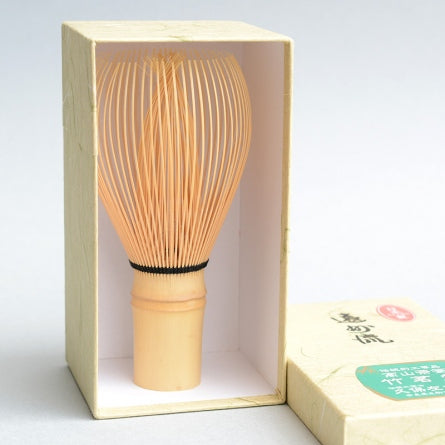The image depicts an intriguing, possibly kitchen-related gadget, predominantly peach-colored with a wisp-like shape, set inside a vertically standing, rectangular box. The box's exterior is adorned with a light yellow hue and subtle gold designs, while the interior is mostly white with hints of pink shadows from the wisp. The wisp itself stands upright, its "fingers" pointing towards the top. Near the base of the fingers is a black circle, leading down to a light yellow handle encircled by a peach band near the bottom.

To the right of the box lies its flat cover, adorned with black foreign characters, likely Japanese or Chinese. This cover also features a light teal patch with additional white foreign characters and a prominent red oval badge with white text in the upper right corner. The background of the image is a predominantly gray tone, casting a shadow to the bottom left and suggesting that the photo is designed for an online marketplace. Despite its precise detailing, the exact function of the gadget remains unclear, adding an element of mystery to its striking presentation.